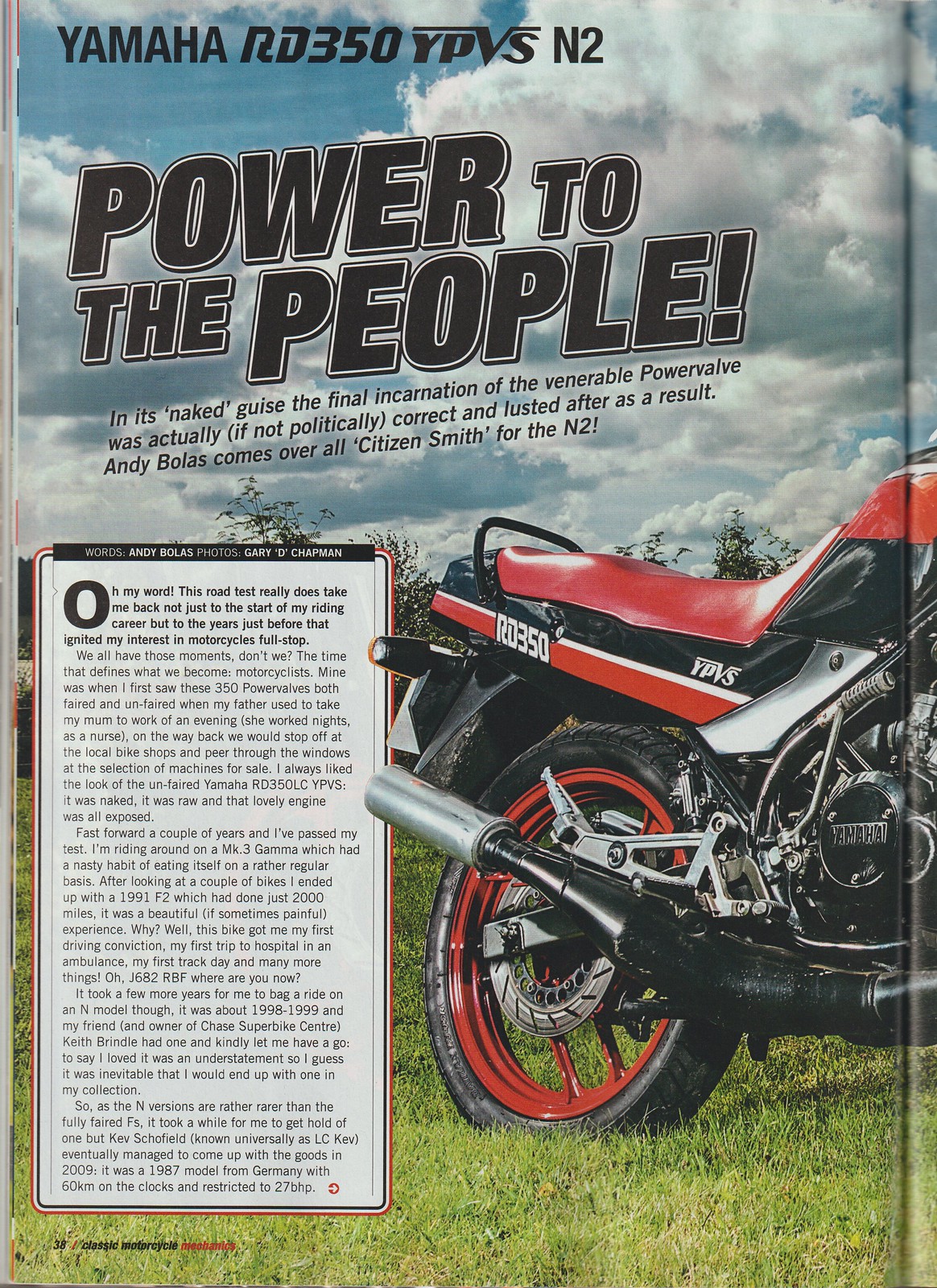This ad poster for a Yamaha RD350 YPVSN2 motorcycle prominently features the slogan "Power to the People!" in large black letters beneath the model's name. Set against a blue sky with billowy clouds concentrated towards the right and lower portions, the visual centerpiece is a sleek red Yamaha motorcycle positioned on green grass. The motorcycle boasts a red leather seat with black and red trim beneath it, while the tank is black with a red stripe. The tailpipe transitions from black to silver at the end, and the wheels have black centers with red rims. In the lower left corner of the photo, there's a rectangular white box containing small, mostly unreadable text with "words: Andy Bolas, photos: Gary Chapman." The image appears to be the left page of a magazine spread, with elements like "a classic motorcycle" and page number "38" faintly visible in the lower left, alongside text like "the final incarnation of the venerable power valve." Overall, the poster merges vibrant design and powerful messaging to capture the essence of the Yamaha RD350 YPVSN2.